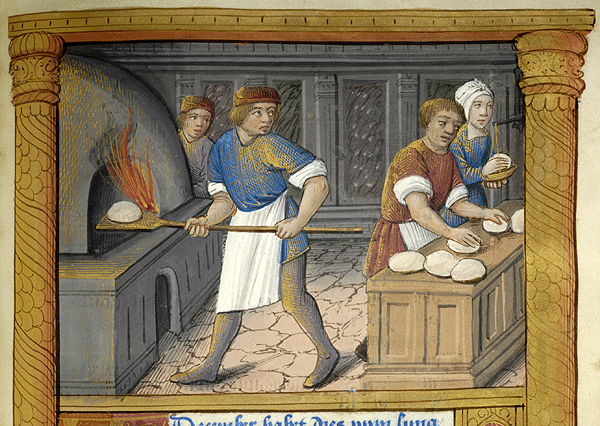The image depicts an old, primitive-style painting framed in light tan wood with intricate etchings, including half circles and lines on the sides and smaller marks on the top. The scene portrays four individuals in a rustic kitchen setting, reminiscent of the Middle Ages, all dressed in attire similar to monks. The central figure, a young man in a blue top and a white apron, is using a long-handled wooden tool to place a pizza or dough into a wood-burning oven. He looks back towards two women who are preparing dough at a station. A fourth person peeks around the corner of the oven, adding to the dynamic atmosphere. Everyone in the painting is gazing towards the right side of the image, as if intrigued or distracted by something off-frame. The painting, which appears to be an illustration captured from a book, also features a partially obscured inscription at the bottom that is not in English.